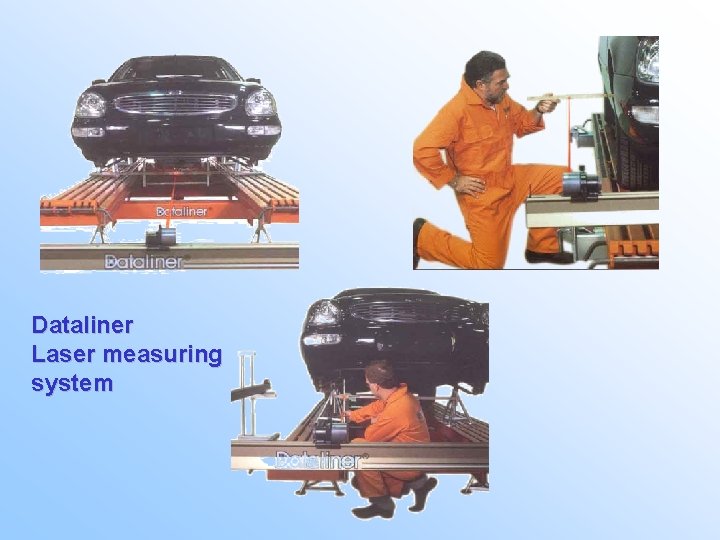The image is a vintage-style advertisement showcasing the "DataLiner Laser Measuring System" against a light blue, almost whitish background. The layout consists of three images: two on the top and one centered below them. In the top left, there is a black luxury car positioned on an orange hoist labeled "DataLiner," appearing to be lifted for inspection. On the top right, a mechanic in an orange jumpsuit, with a device in hand, measures the left side of the car. The bottom image features another mechanic, also in an orange jumpsuit, kneeling beneath the front of the elevated car, utilizing the laser measuring system. Blue text on the lower part reads "DataLiner Laser Measuring System," reinforcing the product's branding and utility for precision automotive work.